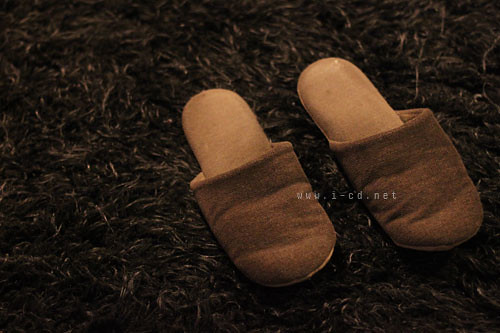The image captures a cozy scene featuring a pair of brown slippers laying on a dark, two-tone shag carpet, blending hues of dark brown and dark green. The slippers, likely meant for indoor use, are slip-on style with no back, designed for comfort. They feature a dark brown, velvet-like material on the outside and a lighter beige cloth on the inside. The slippers, which appear to be the type suitable for a grandparent or dad, show a contrast with their light brown soles. The photo is marked with the website www.i-cd.net, suggesting either the origin of the photo or a place to purchase the slippers.